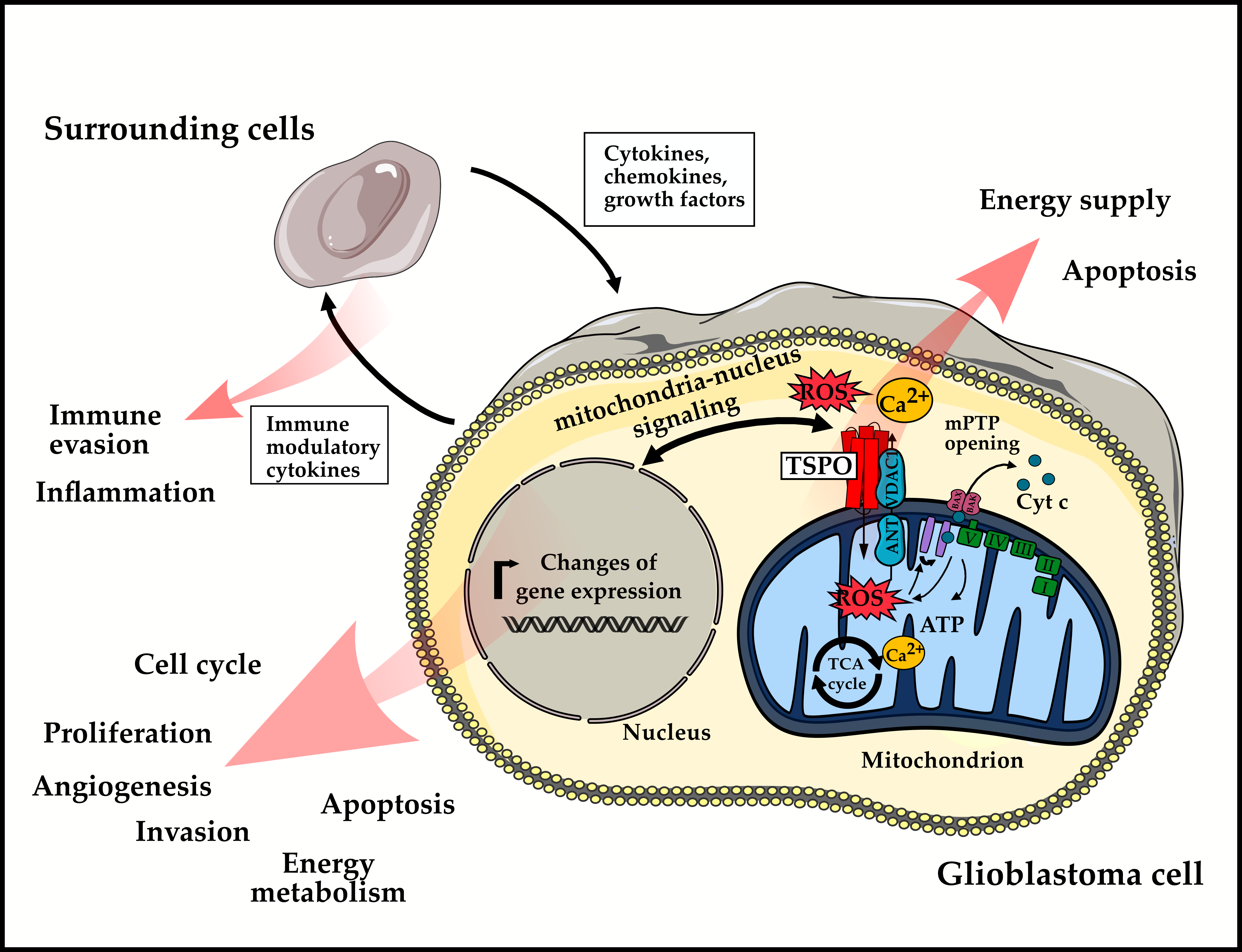This horizontal rectangular diagram depicts a glioblastoma cell and features a white background and a black border. On the bottom right, the cell is labeled as a "glioblastoma cell." The central focus is a detailed cross-section of the glioblastoma cell, allowing us to see internal components like the nucleus and mitochondrion, which are clearly labeled. Arrows and labels annotate various cellular processes, such as "energy supply and apoptosis," indicated by a red arrow pointing upwards, and "cell cycle," with more detailed processes listed underneath. To the left and above the cross-section, there's an illustration of an uncut glioblastoma cell, accompanied by the label "surrounding cells" and further elaborations such as "immune evasion," "inflammation," "immune modulatory cytokines," "cell cycle proliferation," "angiogenesis," "invasion," "apoptosis," "energy metabolism," "changes in gene expression." Additional detailed annotations include "ATP," "TCA cycle," "CYTC," "mitochondrion nucleus signaling," "cytokines," "chemokines," "growth factors," and various other cellular components and processes. This thorough illustration highlights the complex biological mechanisms and impacts of glioblastoma cells, providing significant insights into this formidable cancer.